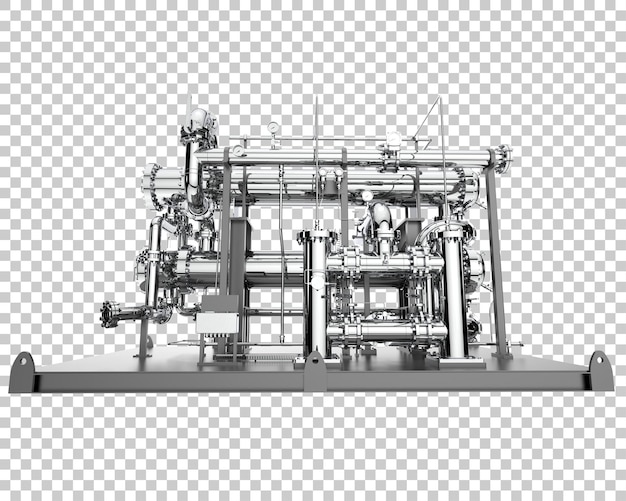This image features a rectangular graphic sample with a gray and white checkerboard background commonly used in digital representations. The checkerboard is composed of many small alternating squares of gray and white. Central to the image is an industrial or printing machine positioned on a steel gray platform. The platform appears to have welded hooks at the corners. Atop the platform is an intricate arrangement of parallel lines or pipes, which intersect with several white-colored pumps positioned underneath the piping system.